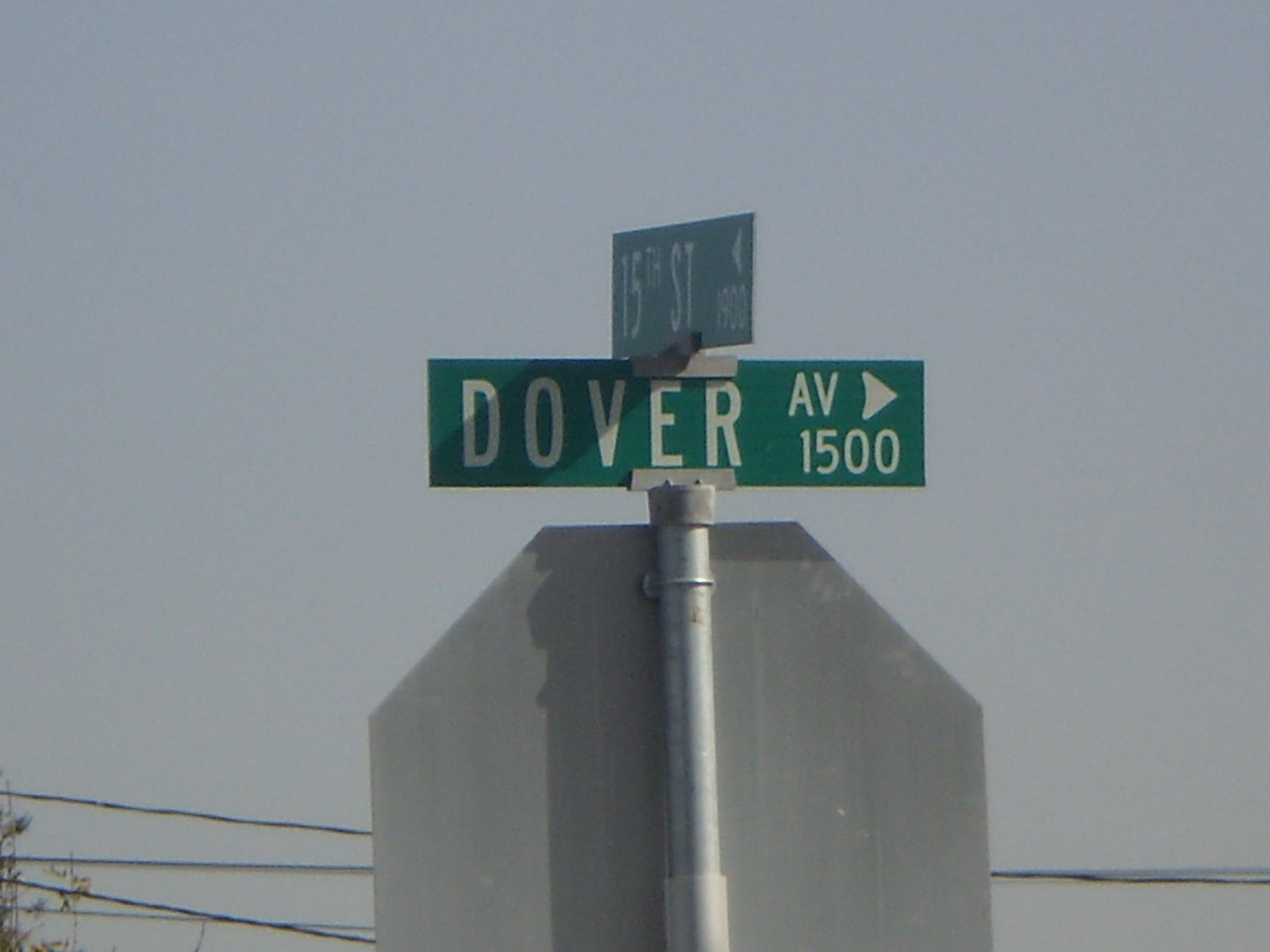This detailed photograph captures an up-close view of an intersection street sign mounted atop a stop sign. The background reveals a gray, slightly hazy sky with some power lines and a bit of a tree encroaching from the bottom left. Dominating the image is the silver back of the stop sign, its octagonal shape clearly visible, though the lower three sides are cropped out of the frame. This stop sign is affixed to a silver-colored metal pole, topped with a small gray knob which holds the street signs.

At the pole’s summit, two green street signs intersect at a 90-degree angle. The lower sign, which is clearly visible, reads "Dover Ave" in all caps, accompanied by a right-pointing filled-in arrow and the number "1500" just below it, possibly indicating ascending street numbers in that direction. Above this, a second street sign labeled "15th Street" extends perpendicularly, with a left-pointing arrow and partially visible number "1900" indicating a different street number sequence. The street signs are securely fastened to the pole with visible U-brackets.